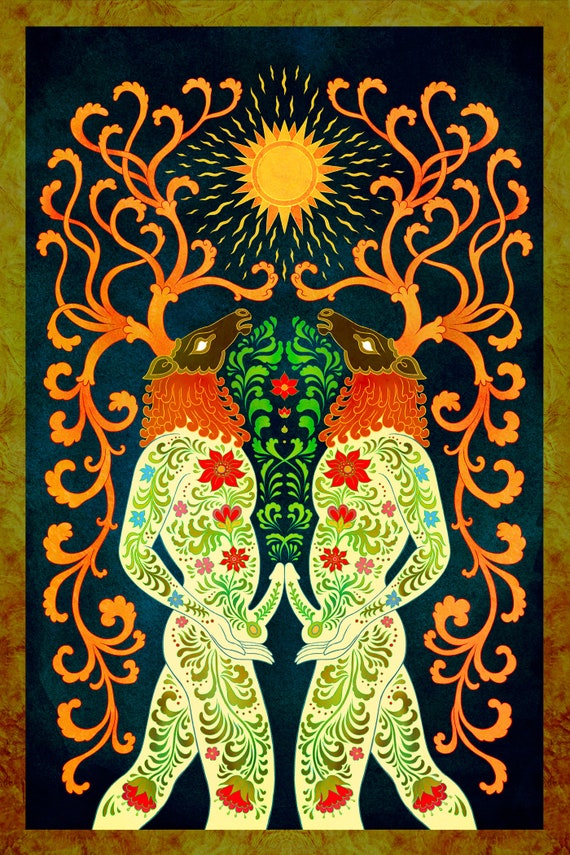The image is a detailed, rectangular drawing, approximately six inches high by three inches wide, bounded by a thin border that transitions from a light greenish-brown at the top to reddish-orange with interspersed striations towards the bottom. Set against a black background that fades to a blotchy blue towards the center, the central focus is on two humanoid male figures facing each other. These figures possess human bodies but have deer's heads, complete with antlers that extend upwards and downwards, forming decorative, vine-like patterns intertwined with leaf-like elements. The deer heads are brown, adorned with red, beard-like fur down the neck. Between the antlers at the top center is an orange and yellow sun with flame-like rays. The bodies of the figures are white, embellished with green vines and red and purple flowers. Their arms are bent at the elbows, with their hands cupping their genitals, while their erections are prominently pressed together.